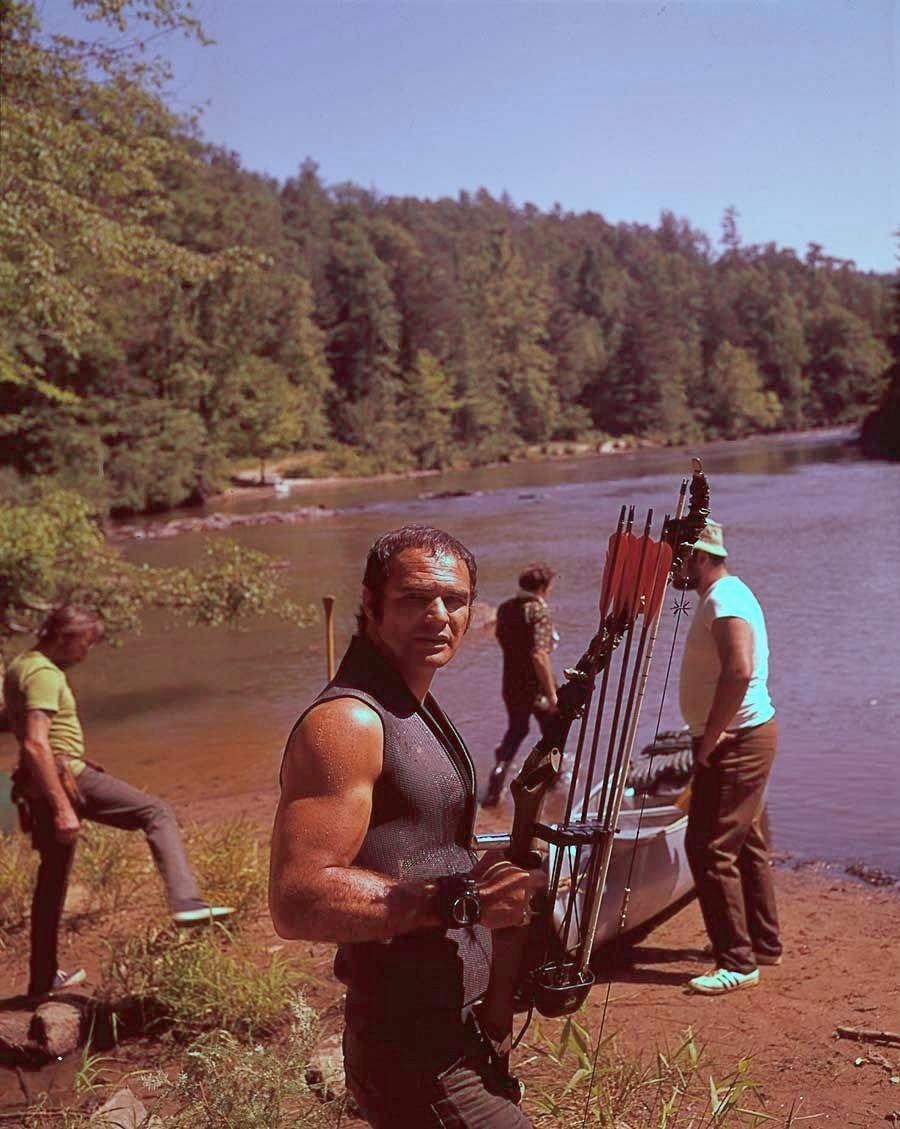This nostalgic image, likely taken in the late 70s or early 80s, evokes a timeless scene set in a picturesque outdoor setting. Bathed in daytime light with clear blue skies stretching horizontally across the frame, the scenery is dominated by a dense forest of trees that transitions seamlessly from left to right. In the foreground, four gentlemen stand poised by the bank of what appears to be a sizable lake or river. A canoe rests on the beach-like shoreline, hinting at their imminent adventure. 

The man at the center, wearing a sleeveless wetsuit and a watch, faces the camera with a confident demeanor, holding a bow and arrow stocked with multiple arrows. To his left, another man clad in a neon green shirt and a belt seems equally prepared, suggesting they are equipped for both fishing and possibly hunting. Scattered around their feet are paddles and various other gear, reinforcing the ambiance of an outdoor excursion.

The layered combination of natural elements and human activity captured in this image embodies a profound connection with nature, harkening back to simpler, rugged times when such outdoor activities were a staple of camaraderie and adventure.